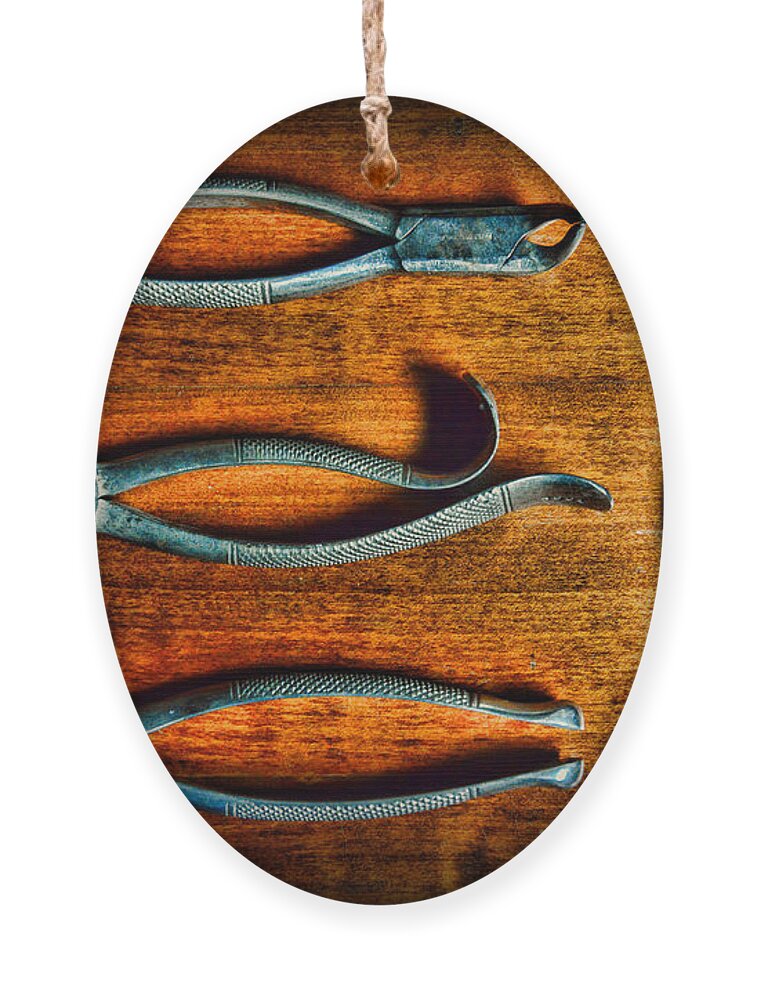The image showcases an egg-shaped, oval pendant made of wood, featuring a visible wood grain design. There is no outer border. At the top, a hole is threaded with a piece of beige twine, suggesting it can be hung. Mounted horizontally across the wooden surface are three old, stainless steel tools, partially cut off at the edges of the oval. The top tool displays handles extending leftward, with the tweezer end pointing right and squared-off tips. The middle tool also shows metal handles, one of which curves upwards. The bottom tool appears to have handles typically associated with a pair of pliers. The tools are predominantly dark pewter in color. The image is devoid of any text, and a variety of earthy colors including white-brown, dark brown, tan, dark gray, and black are present. The photo seems to have been taken in natural setting, providing a clear, detailed view directly at the pendant.